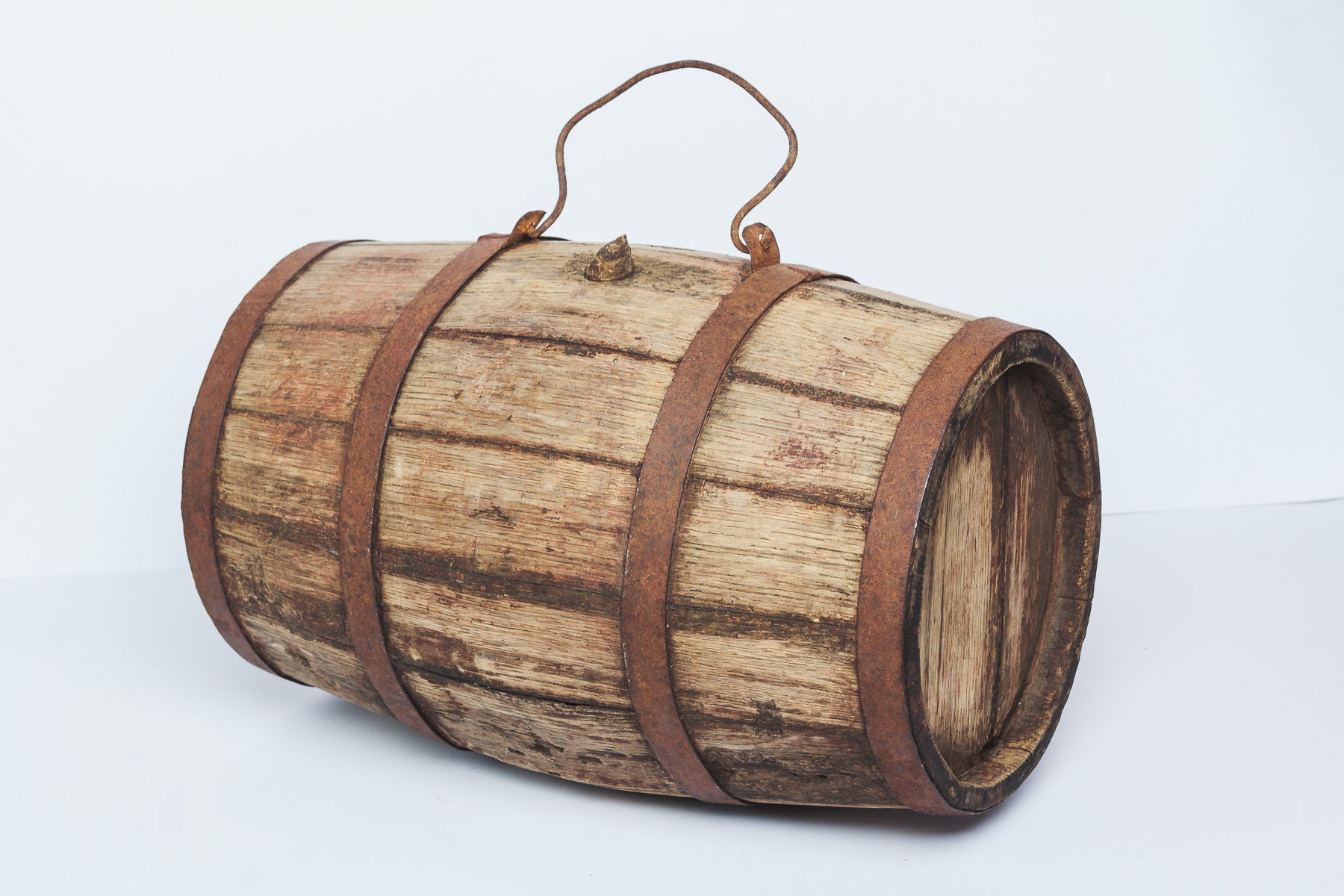This detailed, color illustration features an old oak barrel lying on its side in a landscape orientation against a light gray background. The barrel, crafted from light beige wooden slats, shows signs of aging with much of its original darker stain worn off. Nestled between the slats is a dark brown chinking. Metal bands, likely originally iron, now rusted, encircle the barrel at the ends and spaced evenly around the center. A sturdy, curved metal handle, made from thick wire, is affixed to the top of the barrel between the two center bands. A small knob for a plug is visible between the handle's eyelets. The barrel's front end is directed towards the bottom right of the image, while the back end angles towards the top left. The image, rendered in a 3D style, presents the subject dramatically with no visible text or markings, highlighting the barrel's rustic textures and colors in shades of tan, dark brown, light brown, and hints of black.